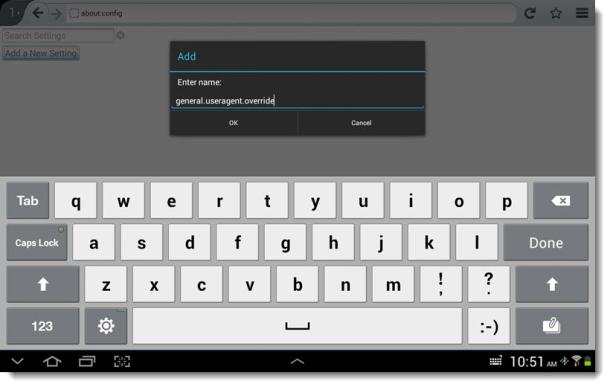The image depicts a horizontally oriented mobile device, likely a tablet or a cell phone, displaying an on-screen keyboard. At the top of the screen, there is a black rectangular notification box with the text "Add and enter name and general agent override, general user agent override" along with options to either "Okay" or "Cancel." 

The keyboard below this box features white keys with black letters, all set against a light gray background. Special keys such as "Tab," "Caps Lock," "Done," and the backspace key are highlighted in dark gray. 

The status bar at the bottom shows the current time as 10:51 AM, alongside icons indicating an active internet connection and a battery level at approximately 50%. In the background, partially grayed out, is a search bar with the text "About configuration," alongside options for "Search settings" and "Add a new setting."